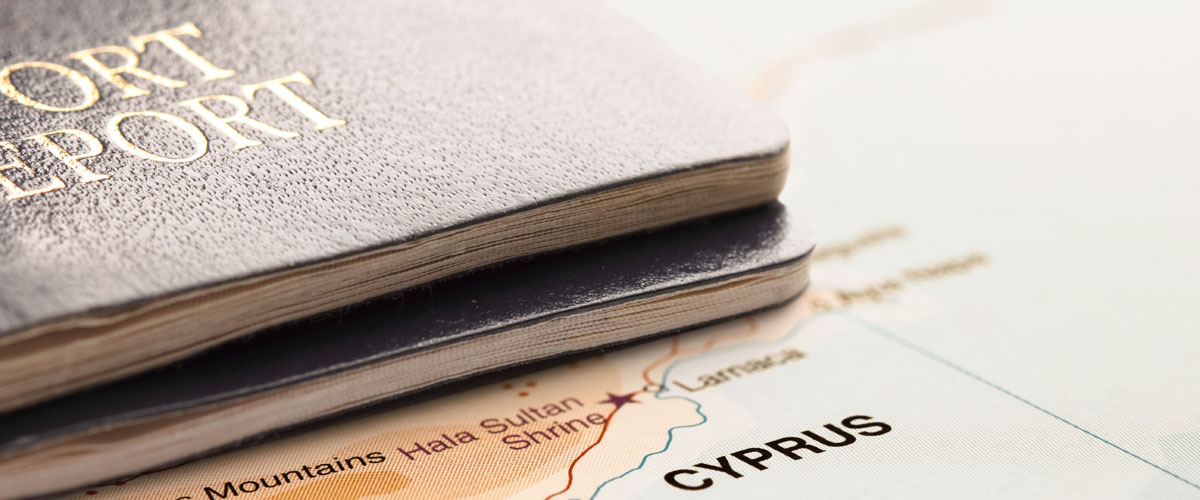In this image, the focus is on a close-up section of a flat-laying map depicting the island of Cyprus, prominently labeled in large, black capital letters against a light blue background, representing the surrounding water. The island itself is shaded in tones of orange and light brown to indicate elevation changes. Key points on the map include the "Hala Sultan Shrine," marked with a red star, and other points of interest like "Mountains" and "La Manca," although some locations are blurred and unreadable.

On top of the map lie two thin, leather-covered books, which appear to be passports. The blue, possibly navy, covers are distinguishable, resembling those typical of US passports but labeled in multiple languages, suggesting they are from a different country. One of the passports at the top is partially visible, showing fragments of the word "PASSPORT" with letters "ORT" and "E-P-O-R-T" in gold print due to the cropping of the image. The compact composition implies a focused presentation, possibly for use in travel-related media.